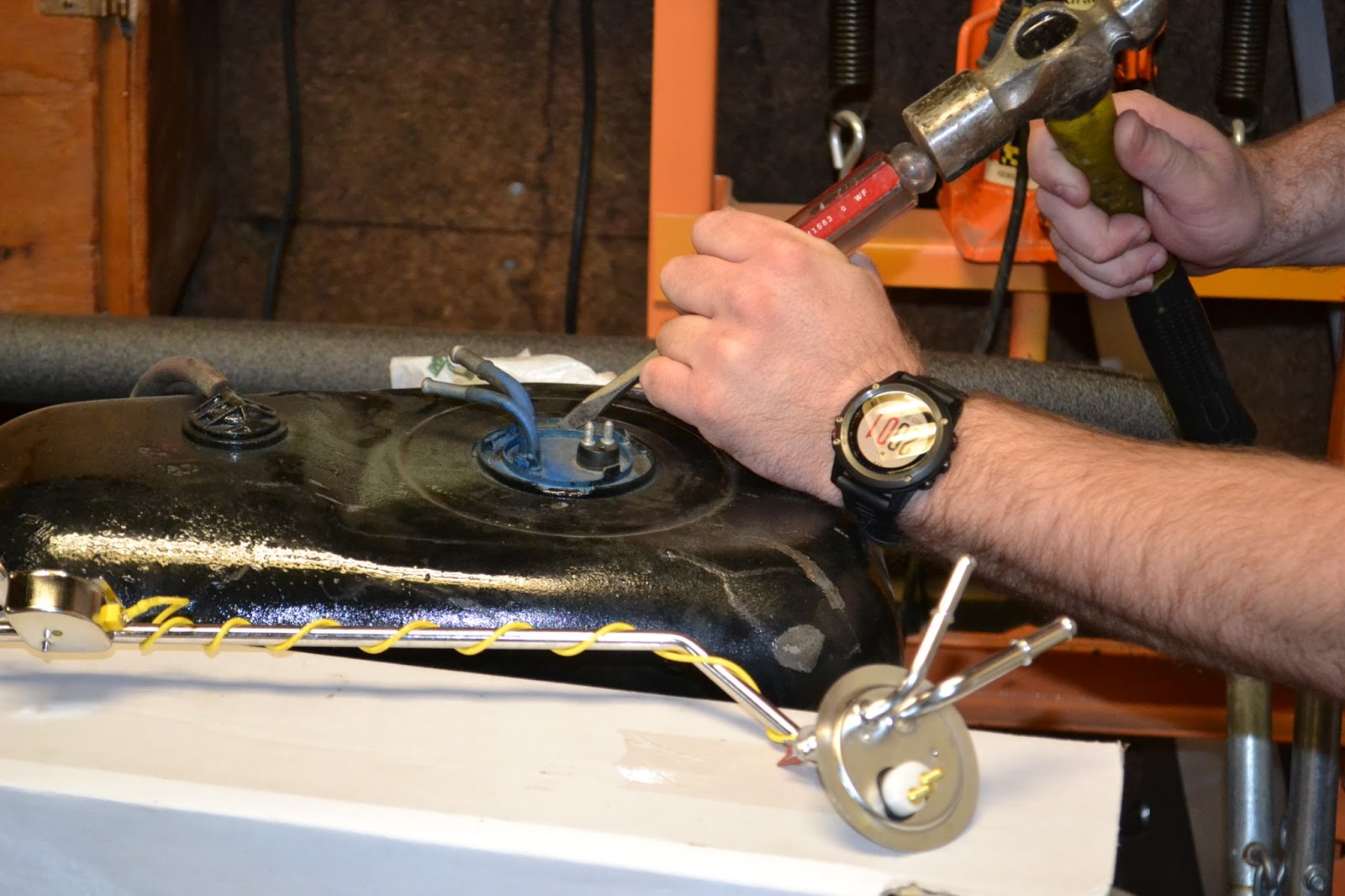In the image, a white Caucasian male is meticulously working on what appears to be a wire or cord. He has a digital wristwatch with a light gray face on his left wrist, displaying the numbers "01" or "10". The man is gripping a tool with a black or dark blue handle and a grayish metal head. This tool appears to be a chisel, though its thickness exceeds that of a standard hammer. Held in his other hand is a metallic, possibly Phillips, screwdriver which he is using to drive into a small blue circular component with two protruding wires.

Behind him is a set of orange shelving units made of what looks like dark brown plywood. Some black object, potentially a drum, is also visible in the background. In the foreground is a silver metal pipe with a circular plate attached to it, resting on a small white countertop.